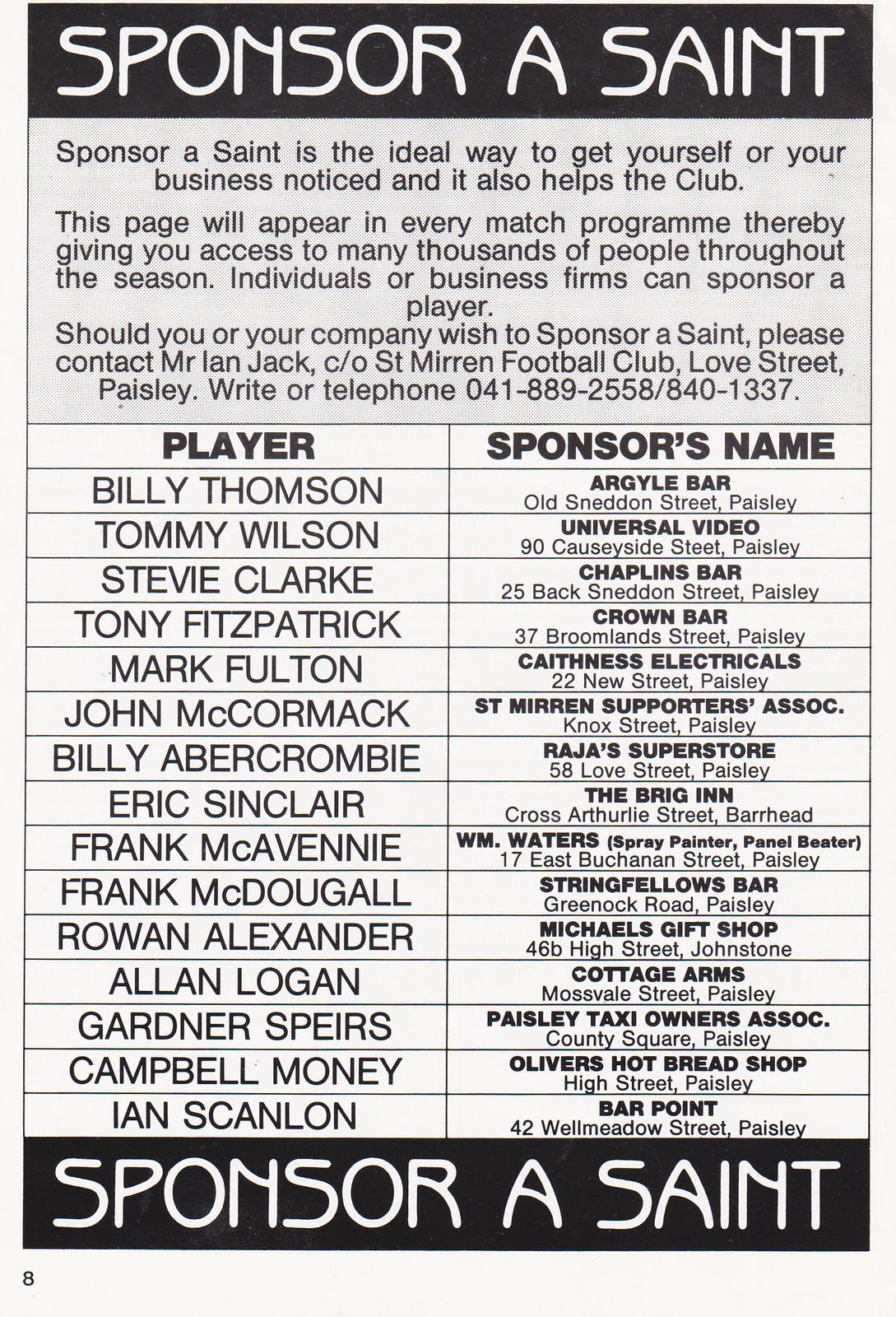The black and white poster prominently features a bold black banner at the top and bottom, both stating "Sponsor a Saint" in white text. Directly below the top header, the poster elaborates: "Sponsor a Saint is the ideal way to get yourself or your business noticed and it also helps the Club." The text continues, explaining that this page will appear in every match program, providing exposure to thousands of people throughout the season. It invites individuals or business firms to sponsor a player, and provides a contact: Mr. Ian Jack, C/O Saint Marin Football Club, Love Street, Paisley, or by telephone at 041-889-255A / 840-1337. 

The main section of the poster displays two columns with headers reading "Player" on the left and "Sponsor's Name" on the right, listing players alongside their respective sponsors. The formatting of the sponsor's information includes the name in bold, with additional details underneath each name. At the bottom, the banner "Sponsor a Saint" repeats, mirroring the top of the poster. It’s a detailed advertisement aimed at encouraging sponsorship to support the club and gain visibility for the sponsors.